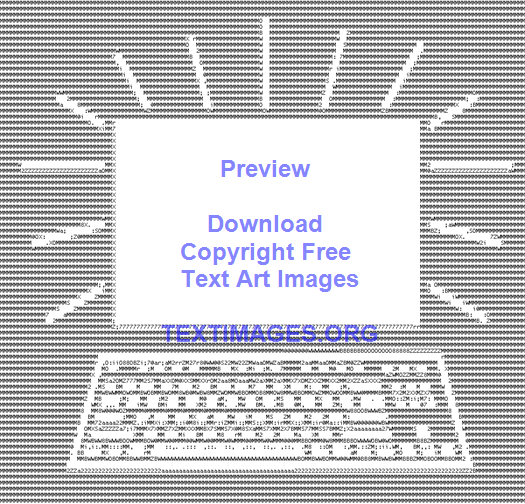The image is a stylized representation of a laptop, meticulously crafted using various keyboard characters. The primary composition consists of a square frame filled with the letter 'P' in alternating patterns, intricately forming the computer's shape. The depiction includes a detailed monitor, key by key on the keyboard, using a range of characters such as semicolons, commas, 'M's, 'D's, and 'O's to represent different keys and functions like the spacebar and shift key. Surrounding the laptop image are white lines extending in various directions to highlight the laptop's form against the black and white pixelated background. The central part of the image features a white box with blue lettering that reads "Preview, Download, Copyright-Free Text Art Images," followed by "textimages.org" in dark blue. The entire image is presented in a cohesive black and white theme, except for the highlighted text in blue, emphasizing its promotional message.